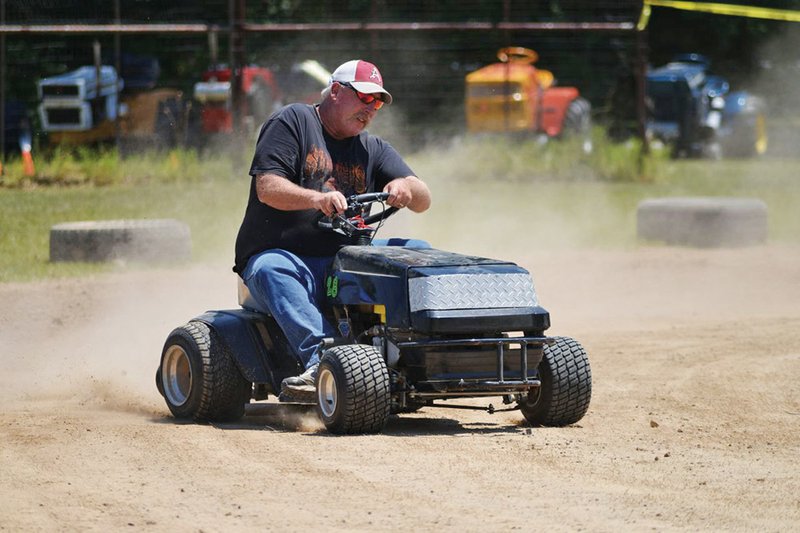In this image, we see a chubby middle-aged man driving a small, go-kart-like vehicle on a beige dirt track. He’s wearing a red and white cap with a white "A" on it, orange sunglasses, and a black shirt with orange accents on the front. He also has on blue jeans and white sneakers. He is hunched over the black steering wheel that appears to be pressed against his stomach, emphasizing the vehicle's small size. The go-kart has a dark blue, dirty front with a silver plate and sits on a flat base supported by three tiny wheels—two in the front and one in the back.

The vehicle is kicking up a dense cloud of dust, creating a foggy atmosphere around the man. In the background, there's a mix of black, blue, red, orange, green, and scattered patches of grass. Additionally, we can see other go-karts and various machinery behind a fence, with what looks like either concrete barriers or old tires. The man, sporting a mustache, appears amused as he steers through the dusty track.